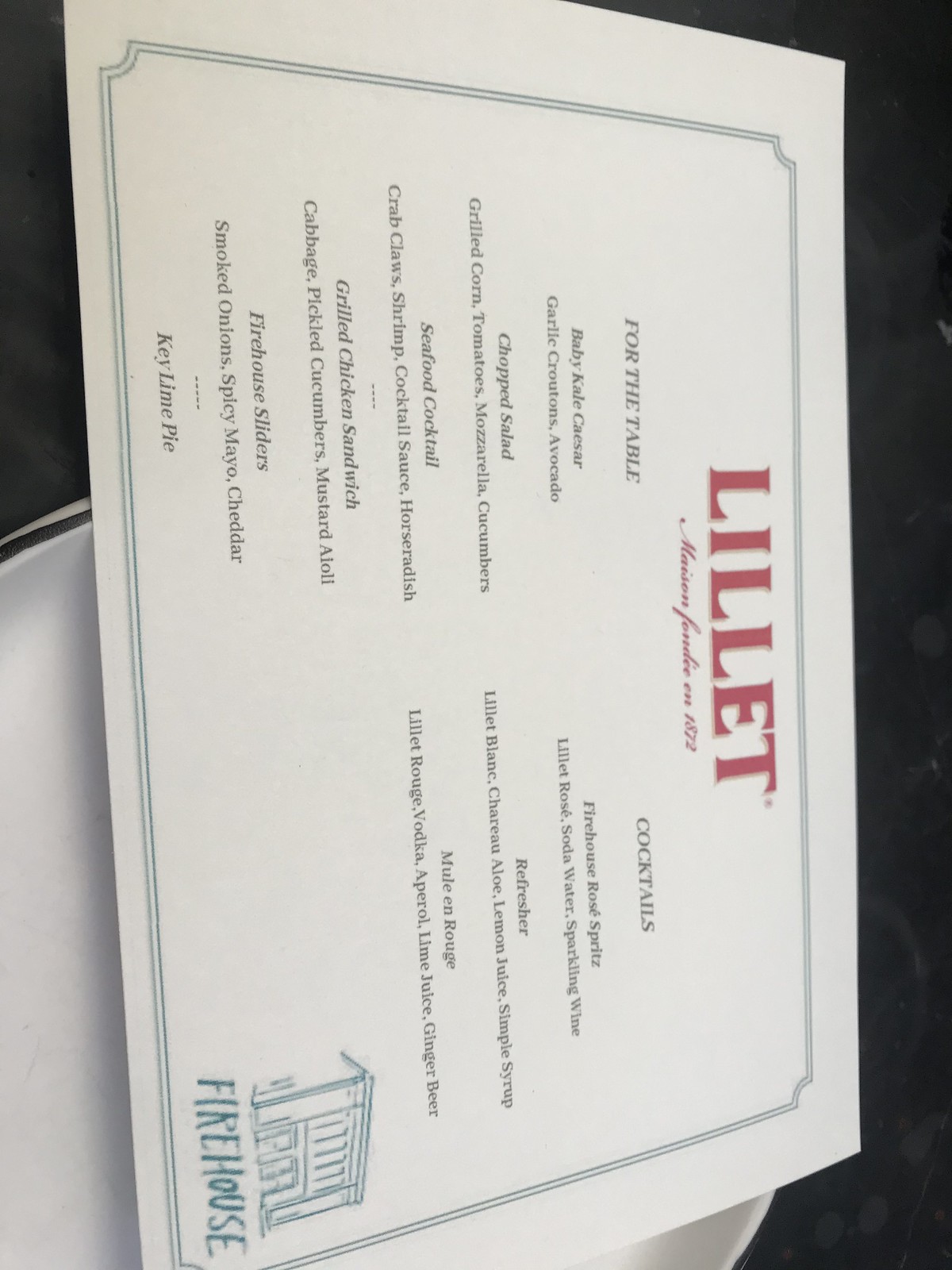This image depicts a vertically-oriented restaurant menu, which is misaligned and facing off to the left rather than directly toward the camera. Set against a dark slate background, the setting suggests the menu may be placed on a slate table or floor. The dark contrast enhances the visibility of the white stock paper of the menu. Behind the menu, there's an ambiguous white object that is not easily identifiable.

The top of the menu reads "Le Lay" and includes the phrase "Mission something in 1872," likely referring to the establishment's history or mission statement. Below this heading, the cocktail section lists various drink options:

- Firehouse Rosé Spritz
- Le Lay Rosé Soda Water
- Sparkling Wine Refresher
- Le Lay Blanc Cheru Aloe Lemon Juice Simple Syrup
- Mule and Rouge
- Le Lay Rouge Vodka Aperol Lime Juice Ginger Beer

Additionally, there is an image of a firehouse, rendered in blue, next to the word "Firehouse." The menu implies that "Le Lay" is probably a winemaker that also offers food at their establishment.